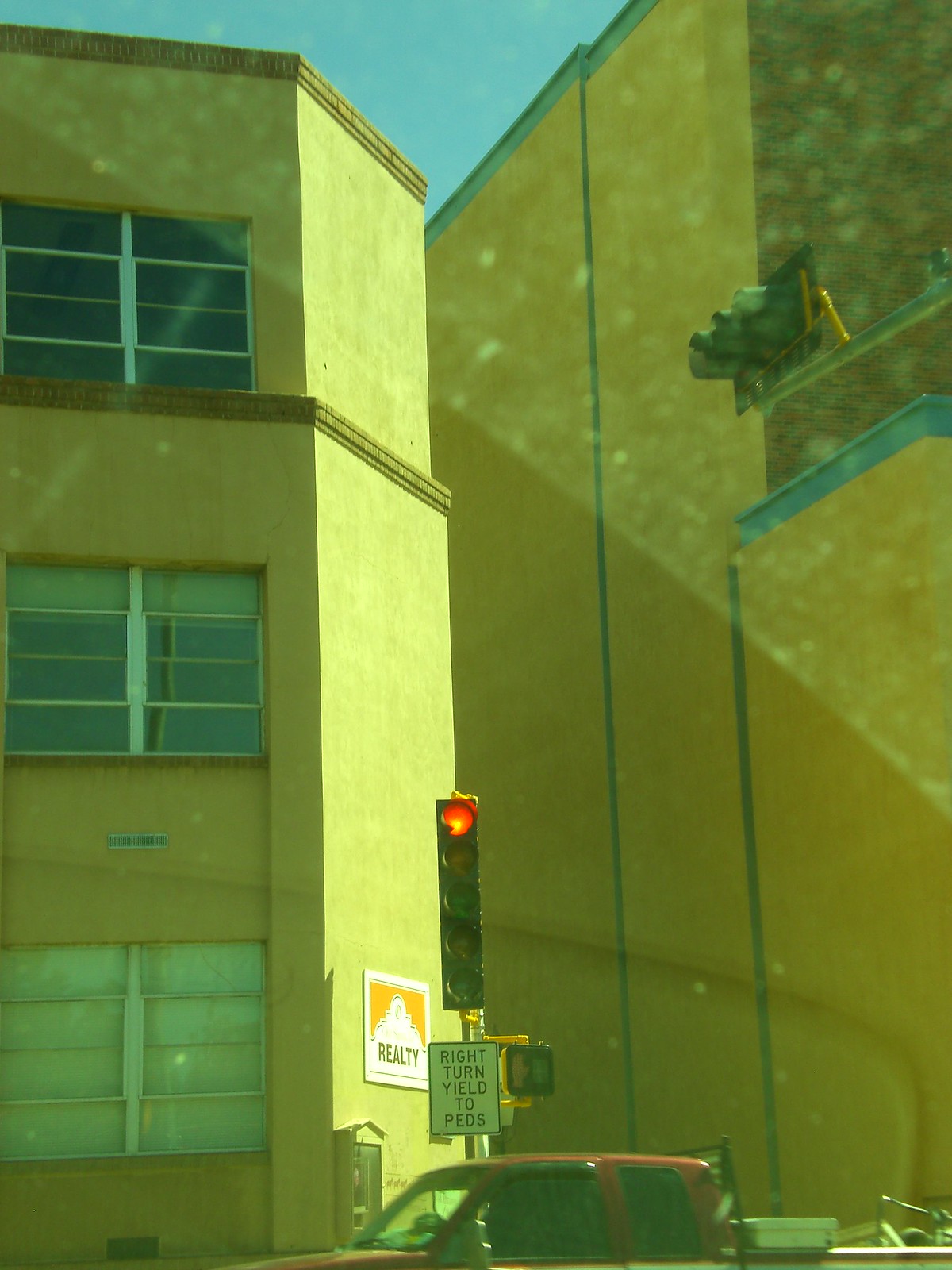From behind a glass surface, likely a window or car windshield, the image captures an urban intersection scene. The foreground reveals the top half of a red pickup truck with an extended cab, its windows tinted or shrouded in darkness, possibly containing a toolbox and some random items in the bed. Above the truck, a traffic light glows red, accompanied by a sign that reads "Right Turn Yield to PEDS." The background features two prominent buildings. The left one is a three-story tan structure with a multi-paneled façade and closed blinds on the lower floor, while open blinds adorn the upper stories, separated by a distinctive ridge trim. This building also has a notable sign that says "Realty," depicting a white mountain against a red background. On the right, a large, windowless building with a yellow wall and green accents forms the other side of the alleyway between them. The sky above is a medium blue, setting a clear yet mundane atmosphere for this city street snapshot.